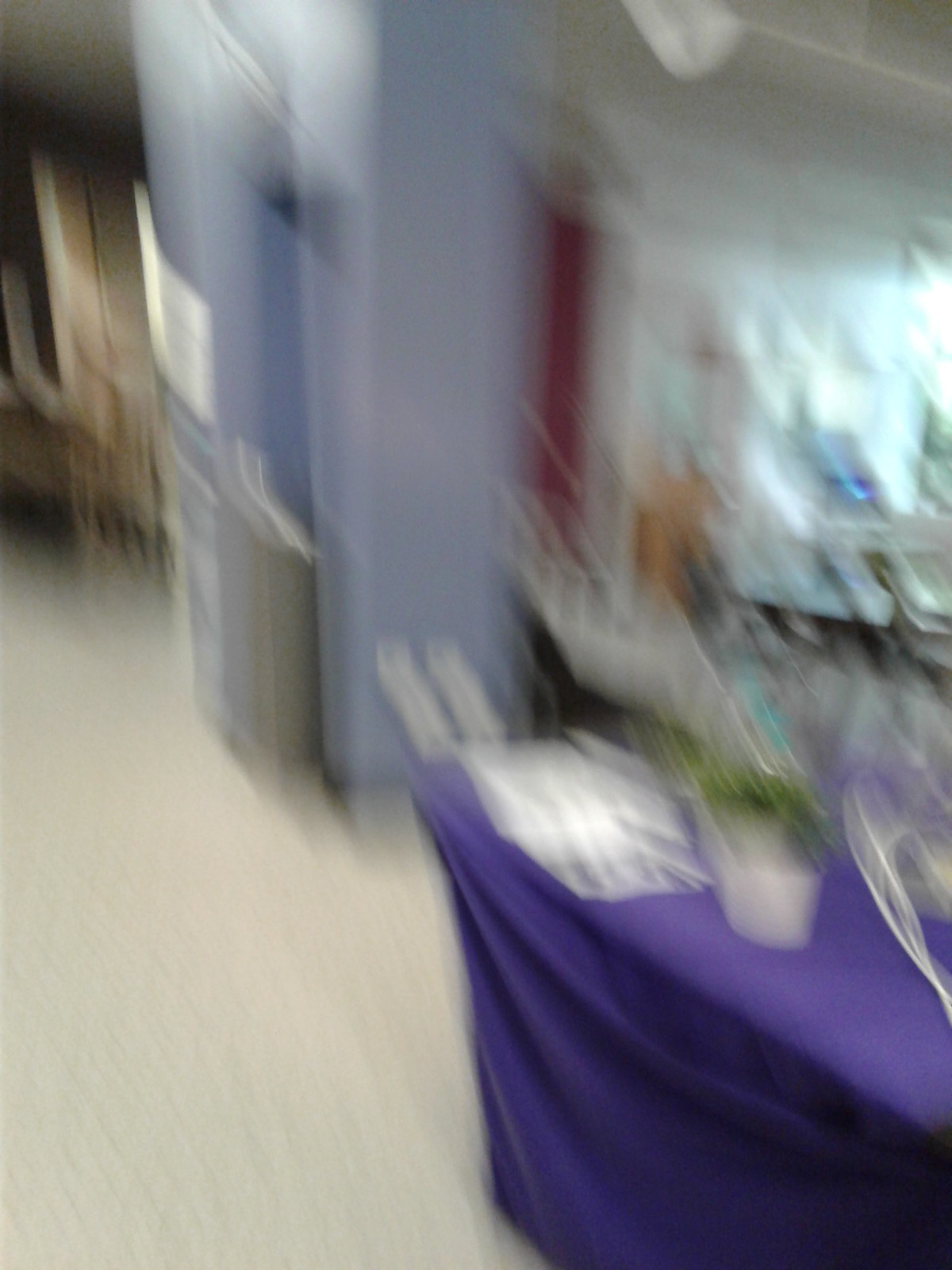This image depicts a highly distorted and blurry indoor setting, making it challenging to discern precise details. In the bottom right corner, a table draped in a purple cloth is notably visible, topped with a white pot containing a green plant, and some additional white items. A large, indistinct blue object occupies the central area of the image, contrasting with the predominantly white floor.

The room features several partially visible elements: white beams stretching across the ceiling, light violet and grayish-blue colored walls, and possibly a red door towards the center. The background includes what appears to be brown chairs and potentially a brown wall or cabinet on the left-hand side near the top, along with windows on the top right, suggesting light filtering in. The overall scene evokes the appearance of an office, a store, or perhaps even a college job fair setup, though the heavy blurring significantly obscures specific details.